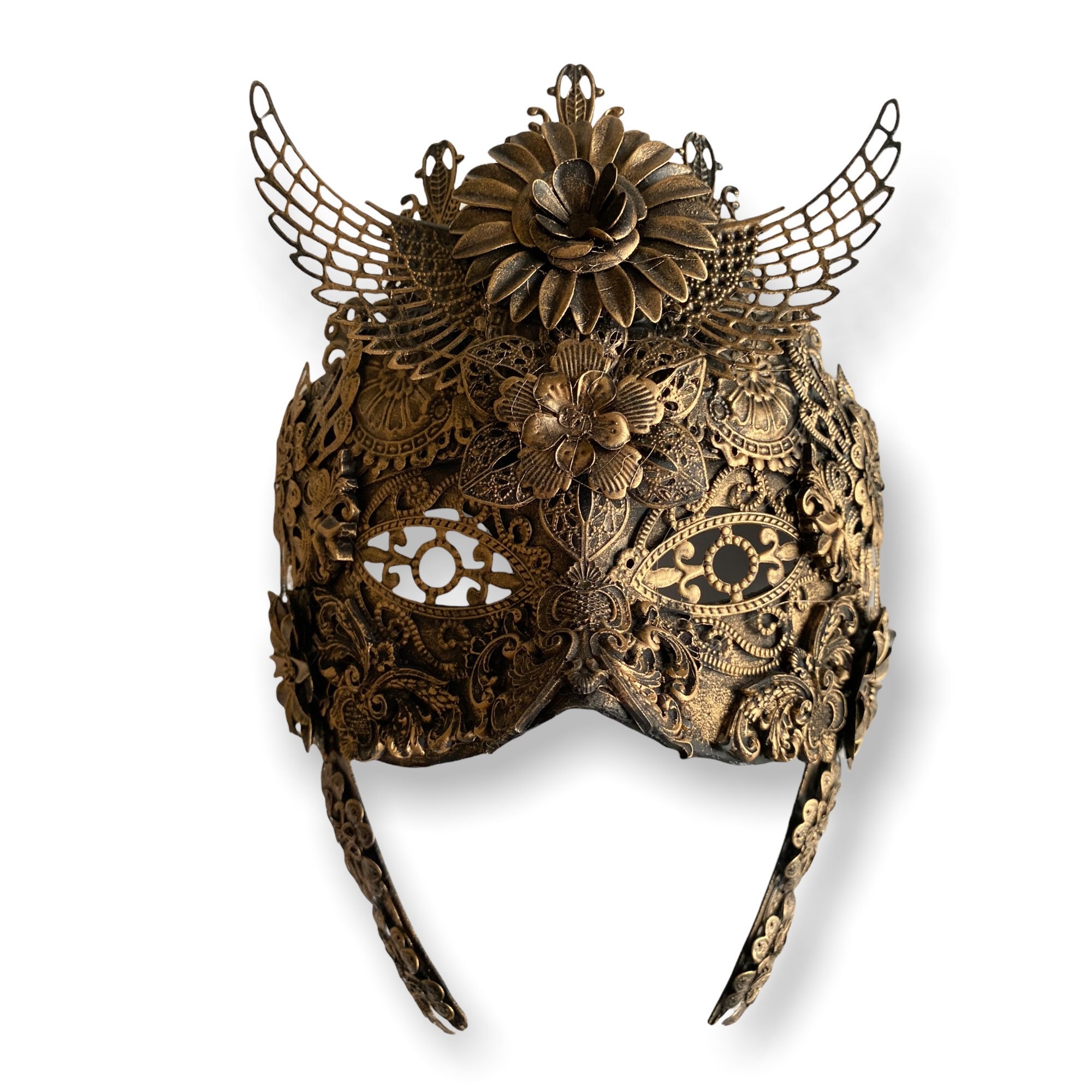This image showcases an intricately designed, traditional-looking mask or helmet, crafted entirely from a brass-like metal. The mask features a pair of elaborate wings on top, shaped with delicate wire that includes ornamental holes. These wings extend out symmetrically to the left and right. Adorning the front is a lotus flower positioned at the top, accompanied by a series of decorative flowers and squiggly lines that cover much of the surface. The eyepieces are particularly notable, each featuring a circle in the center and surrounded by additional ornamentation. One eye appears to be closed, while the other is open. The lower part of the mask includes two ornamental chinstraps hanging on each side. Overall, the mask is richly decorated with fleur-de-lis and flower motifs, giving it a striking and unique appearance.